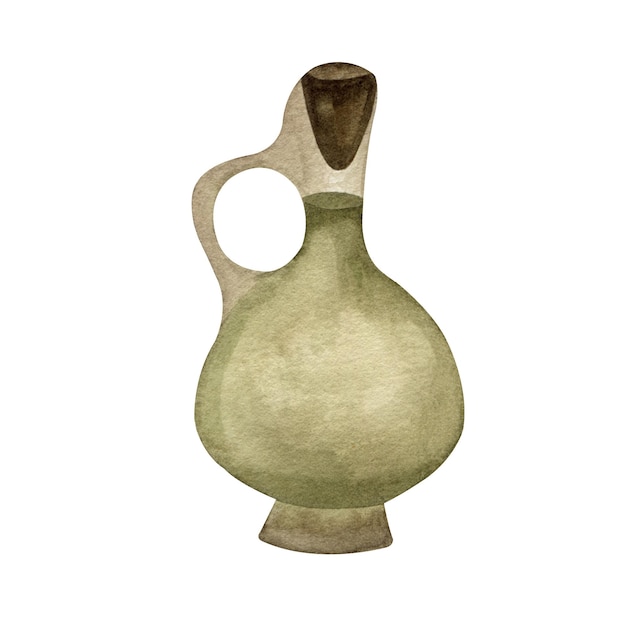The image depicts an old, likely hand-made vase or urn, prominently showcased against a stark white background. The artifact features a rounded, bulbous body colored in olive green, which sits on a smaller, squarish base of a dark brownish-tan hue. The base gradually fades into the green of the main body, creating a harmonious transition. The body of the vase tapers upwards, becoming lighter in color, eventually leading to the neck, where the olive green darkens once more. A notable feature is the handle, constructed from a clear or glass-like material, extending from the main body and curving up to connect to the neck, facilitating easy handling. At the top of the neck, there's a striking dark brown, shark-tooth looking decoration, possibly a cap or cork, which distinctly draws the eye and adds a dramatic contrast. The overall design is both functional and aesthetically pleasing, with a blend of earthy tones and intricate details.